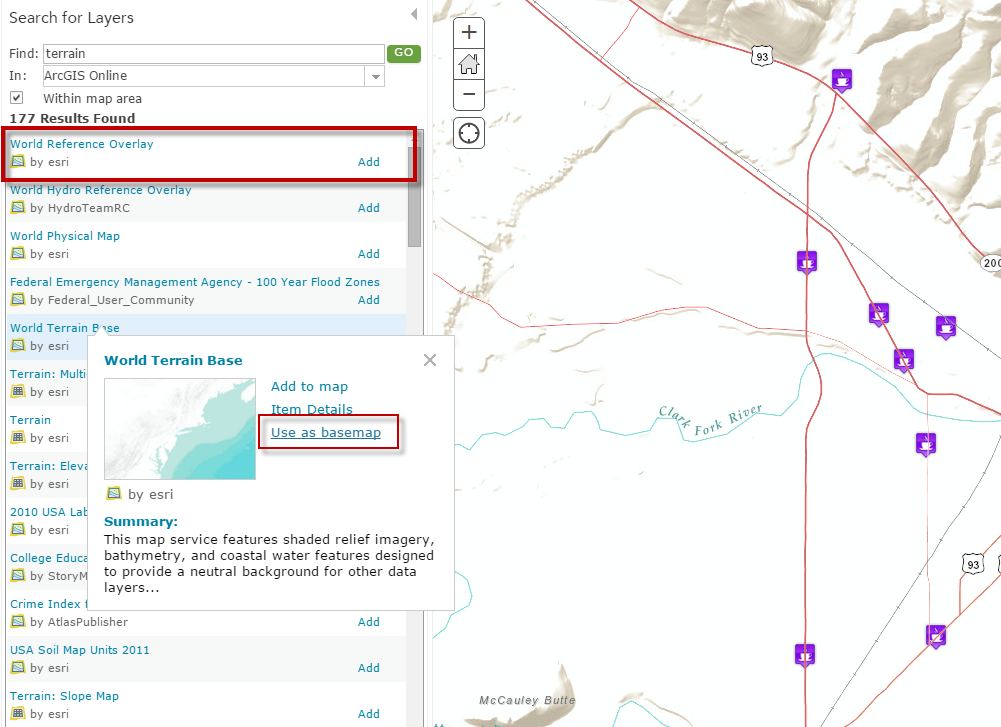This detailed image captures a map prominently featuring the Clark Fork River, which is distinctly marked in blue. The map's color scheme is primarily white and brown. Several red lines with purple icons—each represented by a coffee cup symbol—are scattered throughout the map, numbering around eight in total.

To the left side of the map, a sidebar prominently displays with the title "Search for Layers." This sidebar includes a search input box labeled "Find" and another labeled "In," with the current selection set to "Fine Terrain" in "ArcGIS Online." A checkbox labeled "Within Map Area" is also checked.

The search results reveal that there are 177 items found. The first search result, "World Reference Overlay by Esri," is highlighted with a red box. Every search result includes a title and an author.

Additionally, one search result called "World Terrain Base" is highlighted. This highlighting triggers a small text box with three options: "Add to Map," "Item Details," and "Use as Basemap," the latter of which is also highlighted with a red box. A summary is provided, explaining that this map features shaded relief imagery, bathymetry, and coastal water features designed to provide a neutral background for other data layers. An ellipsis at the end indicates that more information is available.